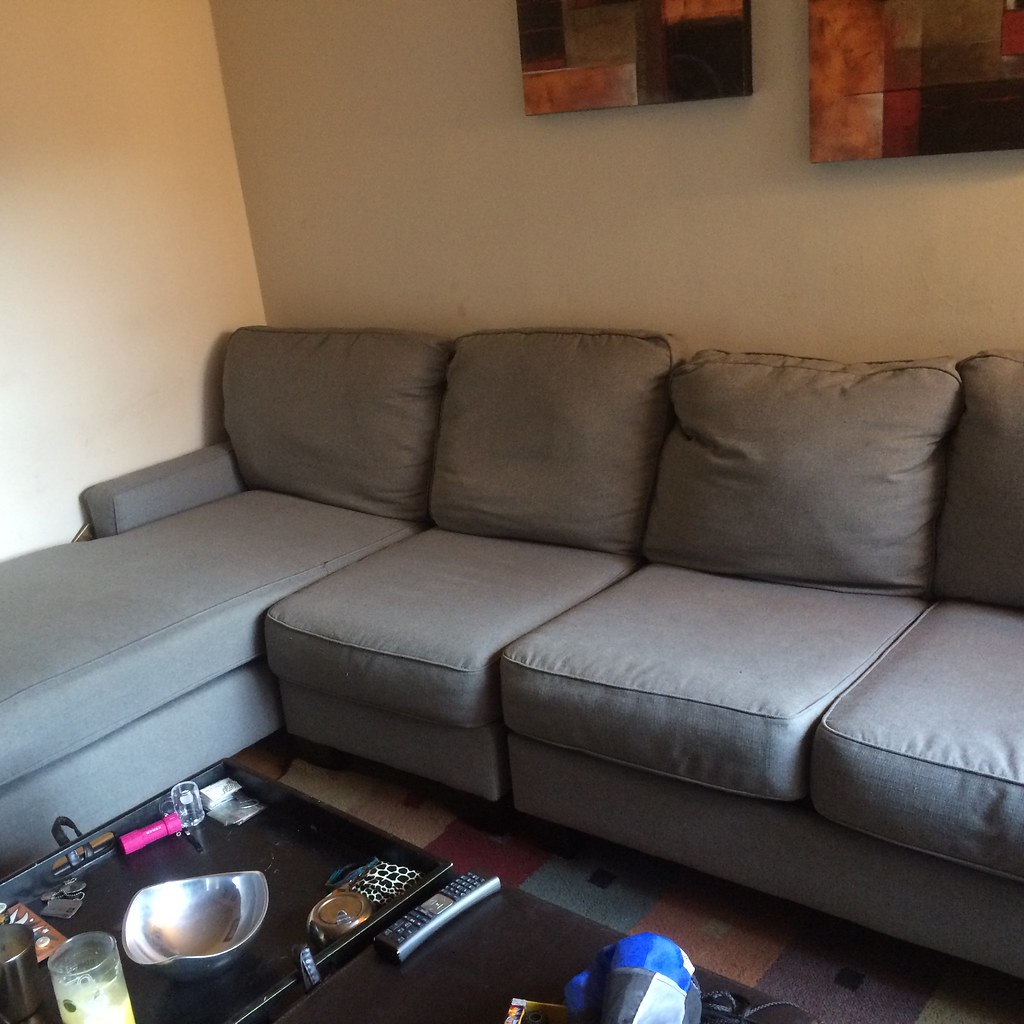This vibrant living room captures a cozy and well-used space, characterized by its light tan, almost beige, walls. The focal point is a comfortable, L-shaped gray sectional sofa occupying the corner; its setup includes three seats on one side and a chaise lounge extending on the other, perfect for reclining or overnight guests. Above the sofa, two abstract geometric paintings in shades of rust, red, dark brown, and light brown add a touch of modern art to the decor.

The floor is covered with a multicolored rug featuring a pattern of large squares with smaller squares in the center, harmonizing with the room’s color palette. Central to the room is a dark cherry-colored wooden coffee table, a bit cluttered with everyday items. These include a black remote control, a silver bowl possibly used as an ashtray, a glass containing a yellowish liquid, what appears to be a pink flashlight, keys, a baseball cap, a white wax candle, and potentially a can of some sort. In addition, personal items like a purse and perhaps a tube of lipstick can be seen, underscoring the room's lived-in charm.